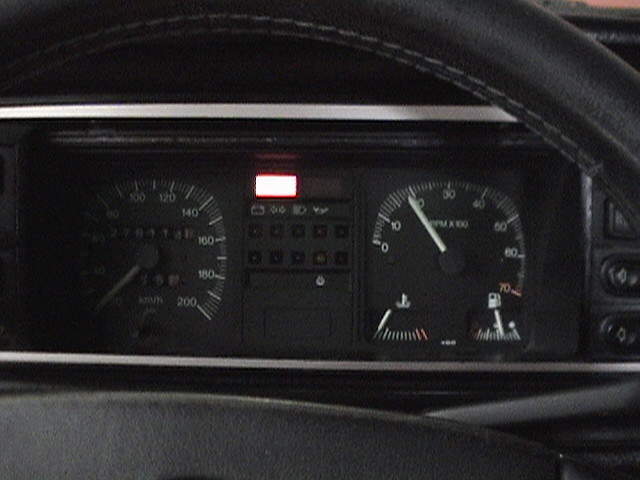A close-up photograph captures the stylish dashboard of a mid-sized to compact car. The steering wheel, made of leather with lighter-colored stitching, is prominently featured in the foreground. The lower portion of the wheel, which is also wrapped in black leather, is just visible at the bottom edge of the image.

Through the steering wheel, we get a clear view of the car's dial-type gauges. On the left, the speedometer ranges from 0 to 200 kilometers per hour, with "KM/H" displayed prominently in white. The odometer below shows a reading of 278,114 kilometers, with the tenth digit not visible in the photograph. The speedometer features a black background with white numerals and a white needle.

To the right of the speedometer is the tachometer, which ranges from 0 to 7,000 RPM. The gauge follows a similar design with a black background and white markings, but the area just under 7,000 RPM is highlighted in red, indicating a critical zone. An oil temperature gauge, marked with an oil can icon, shows temperature from a normal range in white to a critical high in red. The fuel gauge, also with a white-etched scale, is easily identifiable by its gas pump icon.

The dashboard's overall aesthetic is both functional and elegant, with a clear, easy-to-read design that combines practicality with a touch of sophisticated craftsmanship.